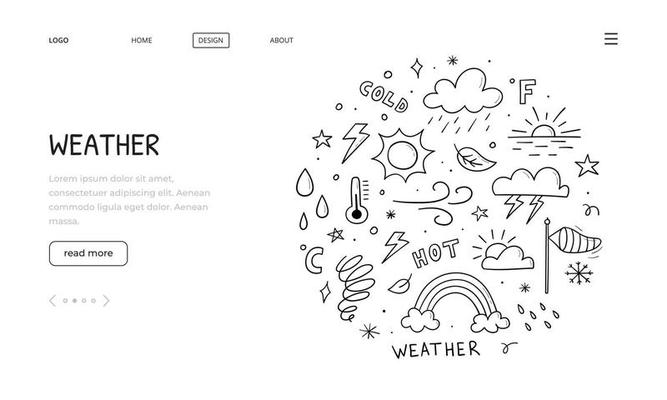The image showcases a monochrome screenshot of a website design interface. The top menu bar includes five options: "LOGO," "HOME," "DESIGN" (currently selected and highlighted with a rectangle), "ABOUT," and a hamburger icon (three stacked lines) on the far right. Beneath the menu, the main content area features the header "WEATHER" in a script-like font, followed by placeholder text, and a prominent curved-edged button labeled "READ MORE." On the right side of the screen, an eclectic collection of weather-related icons and terms are arranged in a circular formation. These include symbols such as clouds, a rainbow, a sun emerging from behind a cloud, raindrops, lightning bolts, thermometers, snowflakes, stars, and other abstract shapes. Words like "COLD," "HOT," "WEATHER," and "F" (for Fahrenheit) accompany the icons. The entire page maintains a minimalist aesthetic with a white background and black graphics and text.